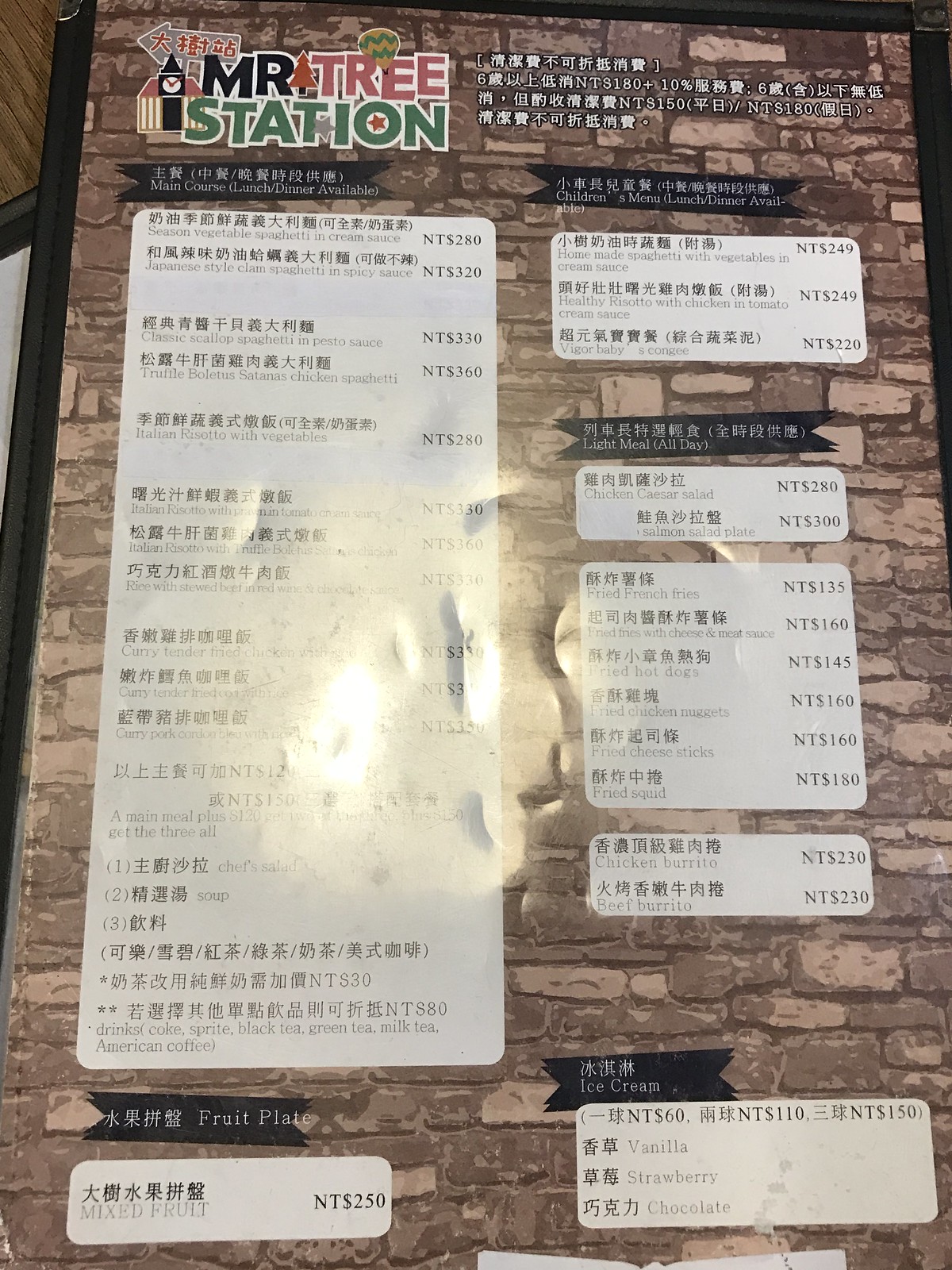This image captures a laminated menu from a restaurant named Mr. Tree Station. The logo for Mr. Tree Station is prominently displayed at the top and features a sophisticated design: "Mr." appears in bold, black block capitals outlined in white; "Tree" is rendered in an orange to brown gradient with white borders; and "Station" is depicted in green, similarly rimmed in white. Notably, inside the "O" of "Station" is a vibrant red star. Nestled between "Mr." and "Tree" is an orange conifer tree with a brown base, paired with a hot air balloon in shades of Dunn and sage green hovering over the "R" and "E" in "Tree." 

To the left of the Mr. Tree Station logo is an illustrative building adorned with a clock resembling a grandfather clock face, with its hand set at 11 o'clock. The menu content is presented in Chinese characters with English translations beneath each item. However, the readability is compromised due to the heavy reflection of light in the center of the laminate, obscuring the text.

The menu’s background is designed to replicate a brick or dressed stone wall, with the stones varying irregularly in shape, size, and color, ranging from Dunn to dark brown hues. Prices are listed in NT, indicating the use of New Taiwan Dollar as the currency.

The menu offers a variety of Western-style options, including fried chicken nuggets, fried cheese sticks, fried squid, chicken burritos, beef burritos, and assorted flavors of ice cream such as vanilla, strawberry, chocolate, and mixed fruit. Beverage options include Coke, Sprite, black tea, green tea, milk tea, and American coffee. Additionally, it features soup, truffle dishes, chicken spaghetti "Santana," and classic scallop spaghetti with pesto sauce.

The menu is slightly tilted, placed on a wood grain table, and the photograph is taken from a downward angle towards the rear of the menu, resulting in a somewhat distorted perspective and proportion.